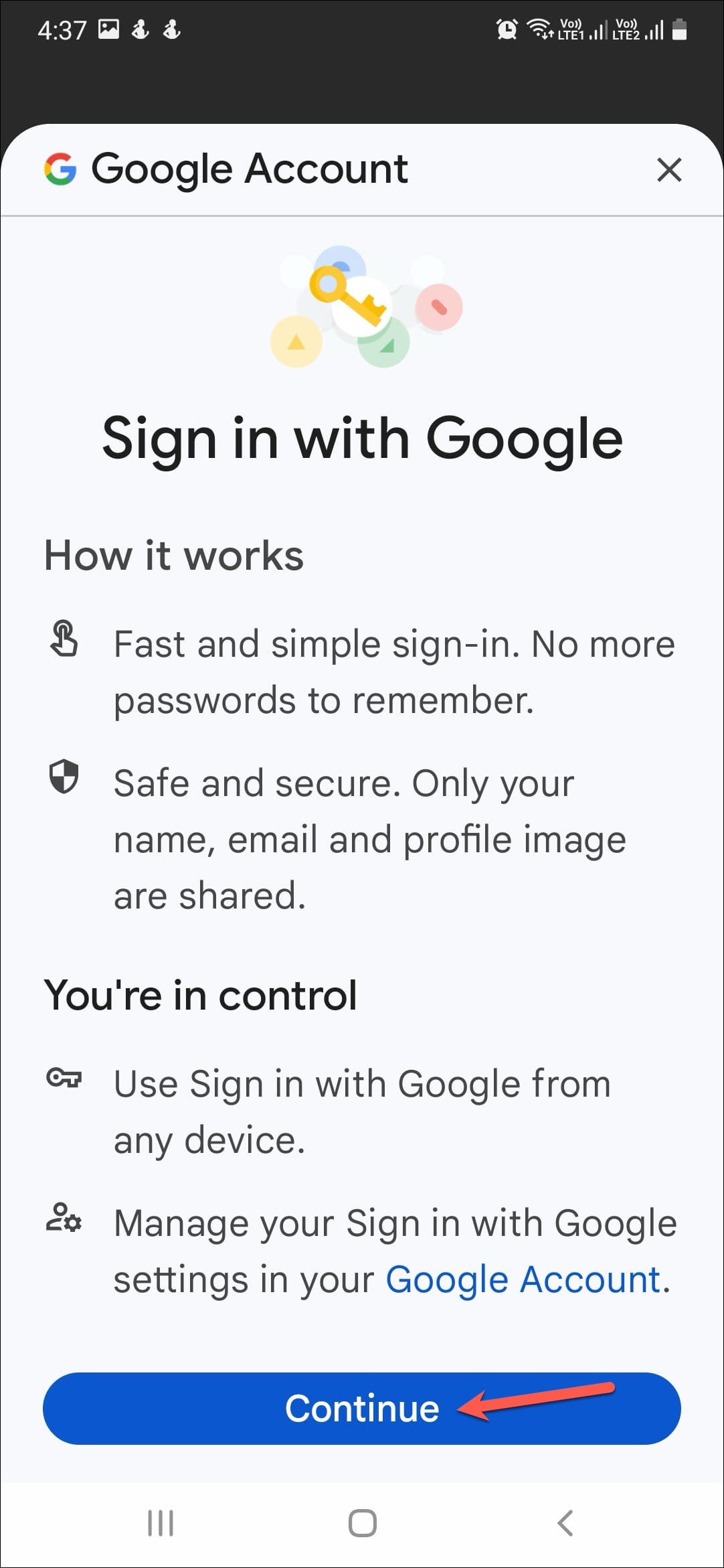The image features a sign-in interface with Google against a white and gray background. The time displayed is 4:37, alongside an image of an alarm clock. A prompt to "Sign in with Google" is displayed prominently, accompanied by a detailed explanation emphasizing the simplicity and security of the sign-in process: "Fast and simple sign-in, no more passwords to remember. Safe and secure, only your name, email, and profile image are shared. You're in control. Sign in with Google from any device."

At the bottom, it encourages users to manage their Google sign-in settings within their Google account, highlighted in blue text. Below, a blue oval button is labeled "Continue" in white text, and a red arrow within a rectangle points towards the "Continue" button, indicating the next action.

Additionally, interface icons are shown along the bottom edge of the image: three vertical lines, a square, and a left-facing arrow, suggesting navigation options or additional settings. This detailed and informative layout assures users of a secure, streamlined sign-in experience with Google.